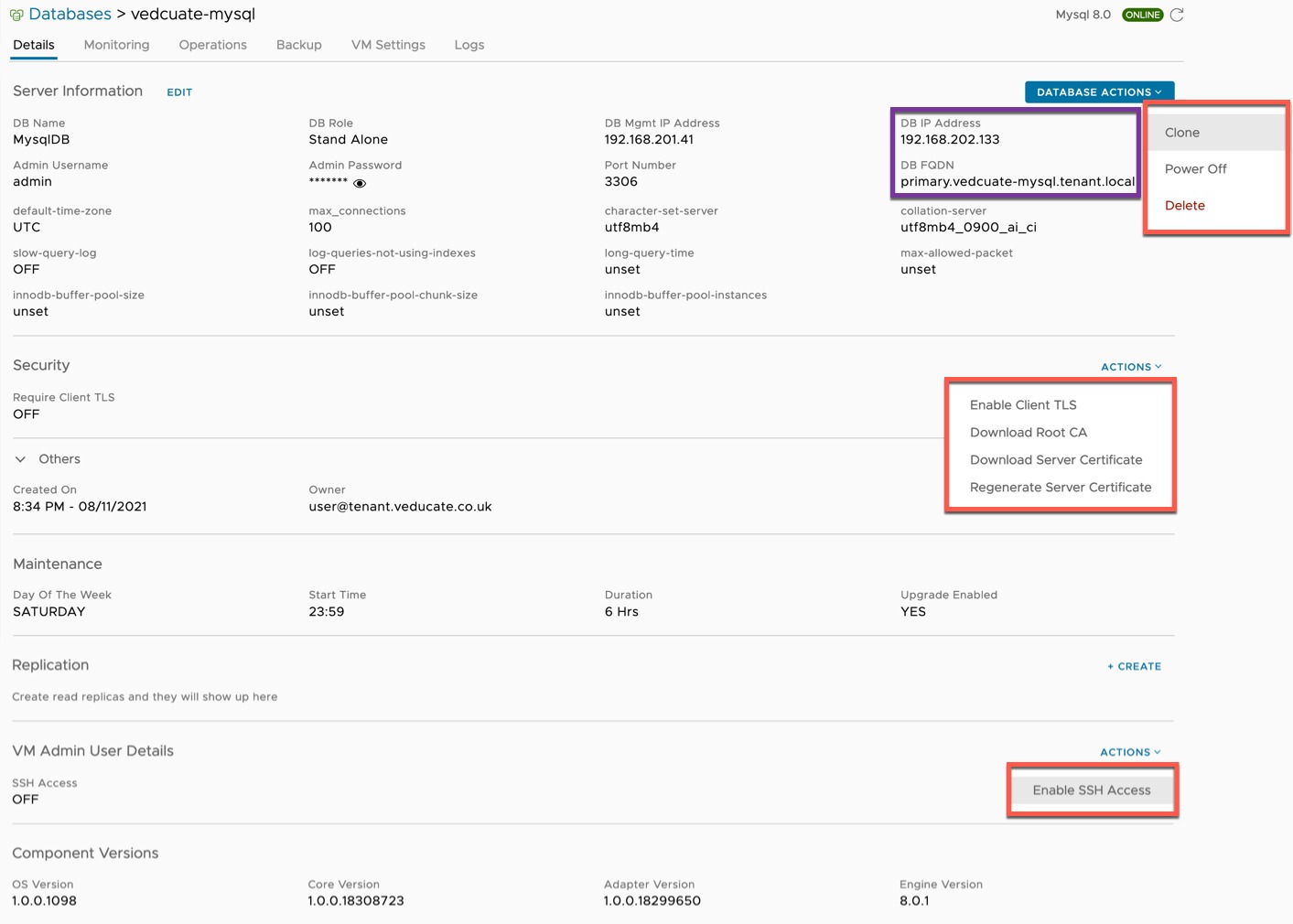**Detailed Description of Database Management Screenshot:**

The screenshot features an interface for managing a MySQL database arranged in a well-organized layout. 

**Top Navigation and Breadcrumb:**
- At the top left corner, there is a breadcrumb navigation trail with a blue background indicating "Databases", followed by black text reading "Regulate-MySQL".
- On the far right, the status of "MySQL 8.0" is displayed beside a green "Online" button and a refresh icon.

**Left-side Menu:**
- A vertical menu bar is situated on the left, listing the following options: "Details", "Monitoring", "Operations", "Backup", "VM Settings", and "Logs".

**Main Content Area:**
- The main content area is divided into seven distinct sections.

1. **Server Information:**
   - This section includes an "Edit" button for configuration.
   - Displays DB name, DB role, and port number (3306).
   - To the right, there is a blue "Database Actions" button.
   - Two parts are boxed in:
     - Purple box: "DB Address" (IP address: 192.168.202.133), and "DBFQDN".
     - Red box: Contains action options - "Clone" (highlighted in gray), "Power Off", and "Delete".

2. **Security:**
   - Indicates "Require Client TLS" is turned off.

3. **Others:**
   - Displays "Create On" date and "Owner" details.
   - A red boxed-in section contains security action options:
     - "Enable Client TLS"
     - "Download Root CA"
     - "Download Server Certificate"
     - "Regenerate Server Certificate"
   - Above this box is an "Actions" dropdown with a down arrow.

4. **Maintenance:**
   - Lists "Days of the Week", "Start Time", and "Duration".

5. **Replication:**
   - Details about replication settings.

6. **VM Admin User Details:**
   - Indicates "SSH Access" is off.
   - To the right, another "Actions" dropdown button is present.
   - Below this, a red box contains "Enable SSH Access".

7. **Component Versions:**
   - Lists versions for "OS Version", "Core Version", and "Adaptor Version".

This detailed description provides a comprehensive view of the functionalities and settings available in the MySQL database management interface.